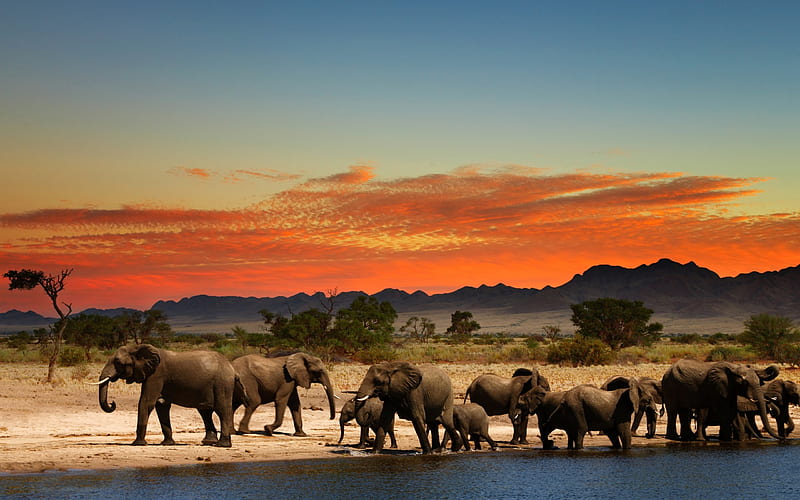The photograph captures a picturesque scene of a herd of elephants gathered at the sandy shore of a body of water, likely a lake or river. The group consists of approximately 10 to 12 elephants, ranging in size from large adults to small babies. Some of the elephants are positioned on the bank while others are partially submerged in the water. The background reveals scraggly trees and bushes, interspersed with patches of grassland, lending an authentic African plains feel to the image. The scene is framed by dark-colored mountains in the distance. The sky above showcases a stunning sunset, with vibrant red-orange clouds melding into a gradually darkening blue sky. One of the trees in the background has a small area of leaves, adding a touch of detail to the landscape. The photo perfectly captures the serene yet majestic atmosphere of these magnificent creatures in their natural habitat as day transitions into night.